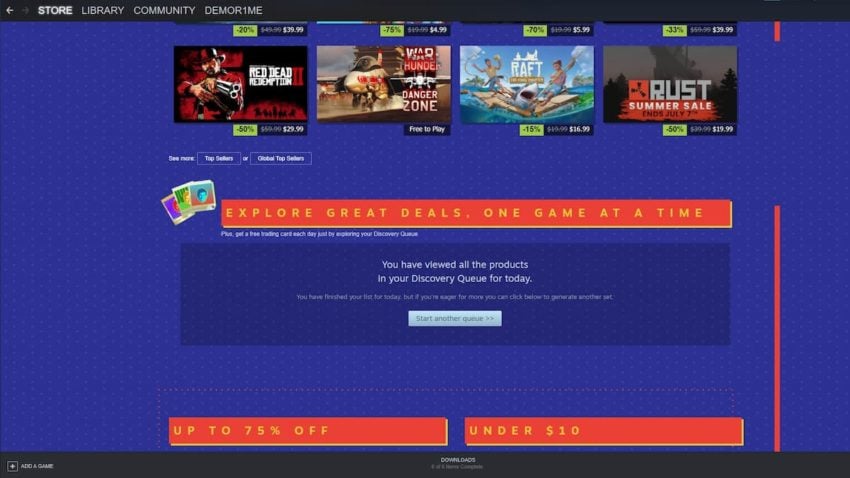This image depicts a computer screen displaying an online video game store interface. The background of the screen features a vibrant gradient of purple and blue hues. There are black horizontal bands at the top and bottom of the screen.

Starting at the top, within the black band, on the left side is a white arrow icon. Adjacent to this icon are several navigation options in white text. The first option, "Store," is bold, indicating it is currently selected. The subsequent options are "Library," "Community," and "demor1me."

Below these navigation options, the main content area is divided into sections, though parts of the images are partially cut off. The upper section showcases pricing information for discounted video games.

1. The first discount box is green and indicates a "-20%" discount with the original price crossed out. The new price is listed in a black box as $39.99.
2. The second box, also green, shows a "-75%" discount. The new price is $4.99.
3. The third box shows a "-70%" discount and lists the new price as $5.99.
4. The fourth green box indicates a "-33%" discount, pricing the game at $3.99.

Below these pricing boxes are images of four video games available for purchase, each accompanied by a name and a brief description:

1. "Red Dead Redemption 2" - Set against a black background, features an image of a man in a cowboy hat pointing a long gun, highlighted by a red background.
2. "War Thunder Danger Zone" - Displays a plane and suggests an aviation theme.
3. "Raft" - This cartoonish image shows two boys on either side of a wooden raft with a shark emerging in the middle, set in the sea.
4. "Rust Summer Sale" - Features a promotional banner with the sale ending on July 7.

Beneath these game images is a bright red bar spanning the screen with orange text that reads, "Explore great deals one game at a time." Directly below this are small white letters on the purple background which mention, "Plus, get a free trading card each day just by [unreadable text]."

Further down, a darker purple section states in white text that, "You have viewed all the products in your discovery queue for today." There's a smaller text beneath, encouraging the user to generate another set by clicking a button. This white button reads, "Start another queue."

At the bottom of the screen are two red panels with orange text indicating additional offers:
1. "Up to 75% off."
2. "Under $10."

Overall, the interface provides a visually engaging layout with detailed pricing and promotional information about the video games.